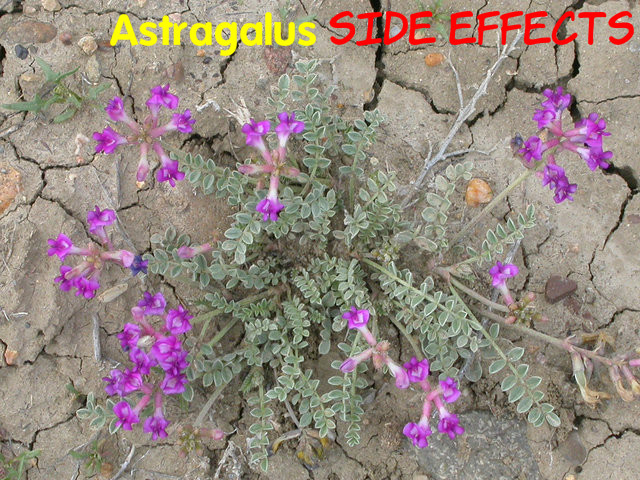This image features a plant identified as Astragalus, which is prominently displayed against a severely parched and cracked earth background. The dry, craggy ground, unable to hold itself together, emphasizes extreme dehydration. The Astragalus plant has silvery-green leaves and striking purple flowers that are small and star-like, radiating outward from slender, green stems. Some descriptions also mention nuances like the flowers having dark pink petals at the tips and being shaped like tiny hollow tubes, adding to their intricate beauty. Nearby, there are scattered brown and beige stones, blending into the rugged terrain. At the top of the image, the text “Astragalus” appears in yellow font, followed by “side effects” in red font, hinting at some caution related to the plant.